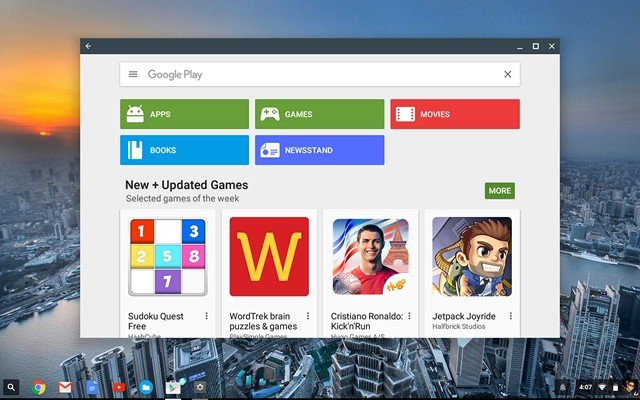The image displays a screenshot of a desktop interface. The wallpaper features a serene sunset over a calm, wavy river bordered by various buildings and apartments, lending a touch of grey to the overall scenery. At the bottom of the screen, there is a taskbar filled with icons for different applications such as a search button, Chrome, email, YouTube, Play Store, and various folders.

A pop-up window for Google Play is open, showcasing the search functionality at the top with the text "Google Play" and three lines indicating options. Below, several categories are displayed: "Apps" indicated by a white robot icon on a green background, "Games" also on a green background, "Movies" on a red background, "Newsstand" on a blue background, and "Books" on a blue background. Additionally, the window highlights a selection of "New and Updated Games."